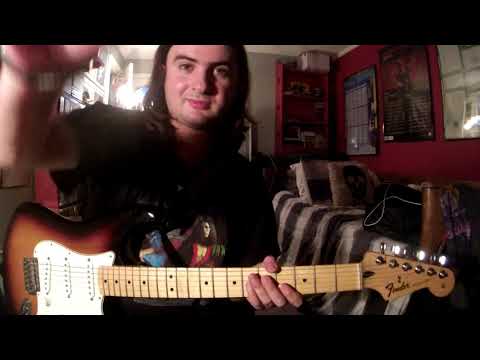In this image, a young man, likely in his mid-20s to early 30s, is captured in what seems to be a screen grab from a YouTube video or a podcast tutorial. He has long, dark hair that falls to his shoulders and is dressed in a black shirt with images of people on it. The scene is set in a dimly lit bedroom with red walls, adorned with various posters and drawings. Behind him, there is a bed with a black and white striped blanket and a skull pillow. He is seated, perhaps in a living or dining area, and is holding a Fender electric guitar that features a combination of brown, black, white, and orange accents with silver knobs. The frame of the photo is rectangular with black borders at the top and bottom, emphasizing the captured shot. The man’s body and face are somewhat backlit, casting parts of him in shadow, while his right hand moves towards the camera, possibly adjusting it.